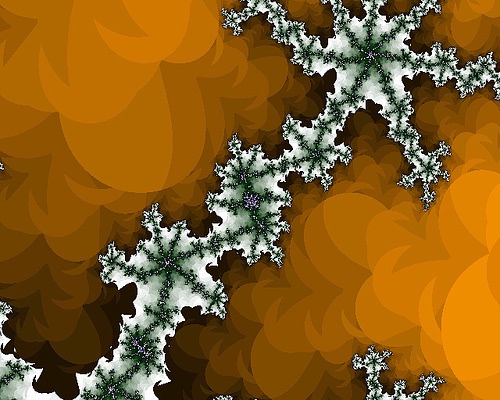The image features an abstract design reminiscent of a Christmas card, with an artsy and intriguing composition. Dominating the center is a network of white, crystalline patterns that resemble elongated and interconnected snowflakes or star-like shapes. These intricate forms crisscross the image, running diagonally from the lower left to the upper right, adding a geometric, almost jewelry-like aesthetic.

The background contrasts sharply with this white, crystalline network, featuring a vibrant orange hue populated with circular, spotlight-like or confetti light patterns that lend a dynamic sense of depth and texture. These circular elements evoke the sense of a festive atmosphere, while the orange swirls and leafy shapes provide a rich backdrop that complements the foreground intricacies.

Overall, the composition blends the delicate, interconnected white patterns with a colorful and lively orange background, creating an evocative image that captures the eye and invites a sense of wonder, much like a unique and unconventional holiday greeting card.